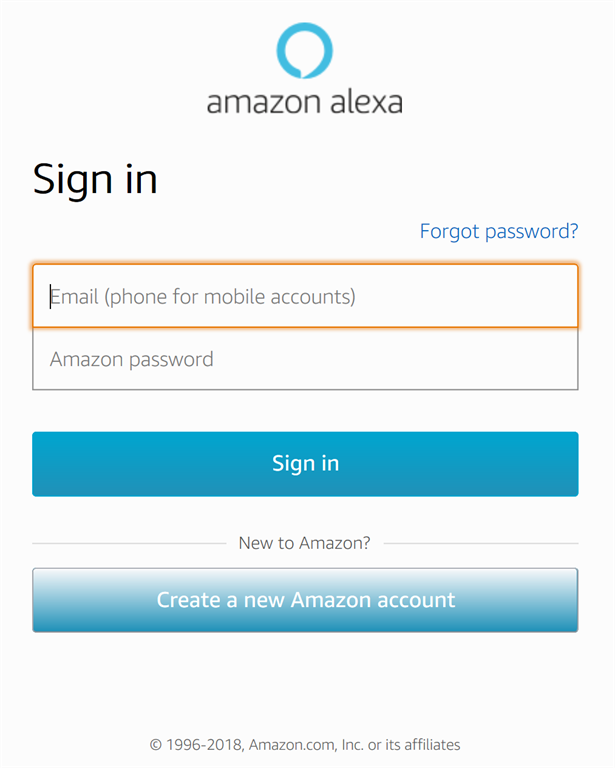The screenshot depicts the Amazon Alexa sign-in page, featuring a clean, white background. Centered at the top, the text "Amazon Alexa" appears in a grey, lowercase font, accompanied by the Alexa logo above it—a white circle outlined in blue, with the pointed end of the outline visible at the bottom right.

On the left side, the word "Sign-In" is displayed in grey. Below this title, there are two input fields: the first labeled "Email (phone for mobile accounts)" and the second "Amazon password". To the right of these fields, "Forgot password?" is written in blue, indicating a clickable hyperlink.

Under the input fields, a blue rectangle button labeled "Sign-In" is prominently displayed in white font. Beneath this button, the text "New to Amazon?" invites new users to create an account. 

Below the invitation, another blue rectangle—featuring a gradient from lighter at the top to darker at the bottom—offers the option to "Create a new Amazon account" in white font.

At the very bottom of the page, the copyright notice "© 1996–2018 Amazon, Inc. or its affiliates" is printed in a light grey font.